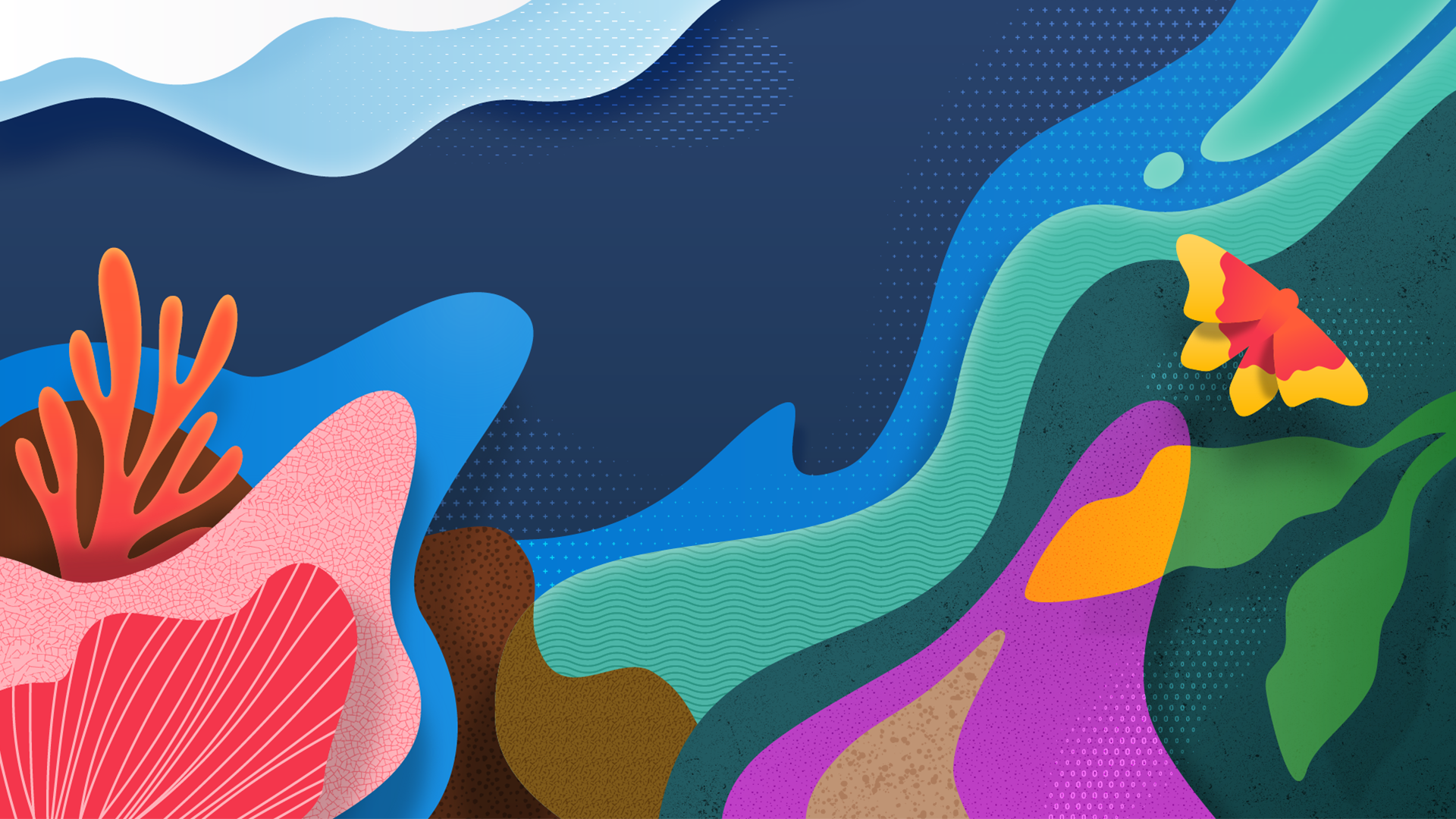This image is a horizontally-aligned, semi-abstract, and colorful digital illustration with cartoonish and stylized elements. The background features interwoven, multicolored waves, starting with white in the upper-left corner, transitioning to light blue, dark blue, and then a mix of seafoam green, dark green, purple, brown, and orange. 

A large blue wave with a lighter blue counterpart spans the left side, with a dark brown hill and vivid coral elements in pink and coral colors situated in the lower-left corner. These coral shapes include intricate, striated pink patterns with thin white diagonal lines.

On the right side, prominently placed, is an orange butterfly with a red or pink center and yellow accents on its wings. The royal blue wave traverses the top-right corner downward towards the middle, providing a dynamic backdrop for the butterfly. The image overall is richly detailed, showcasing a vivid, colorful composition of overlapping curves and shapes with a blend of natural and abstract art forms.